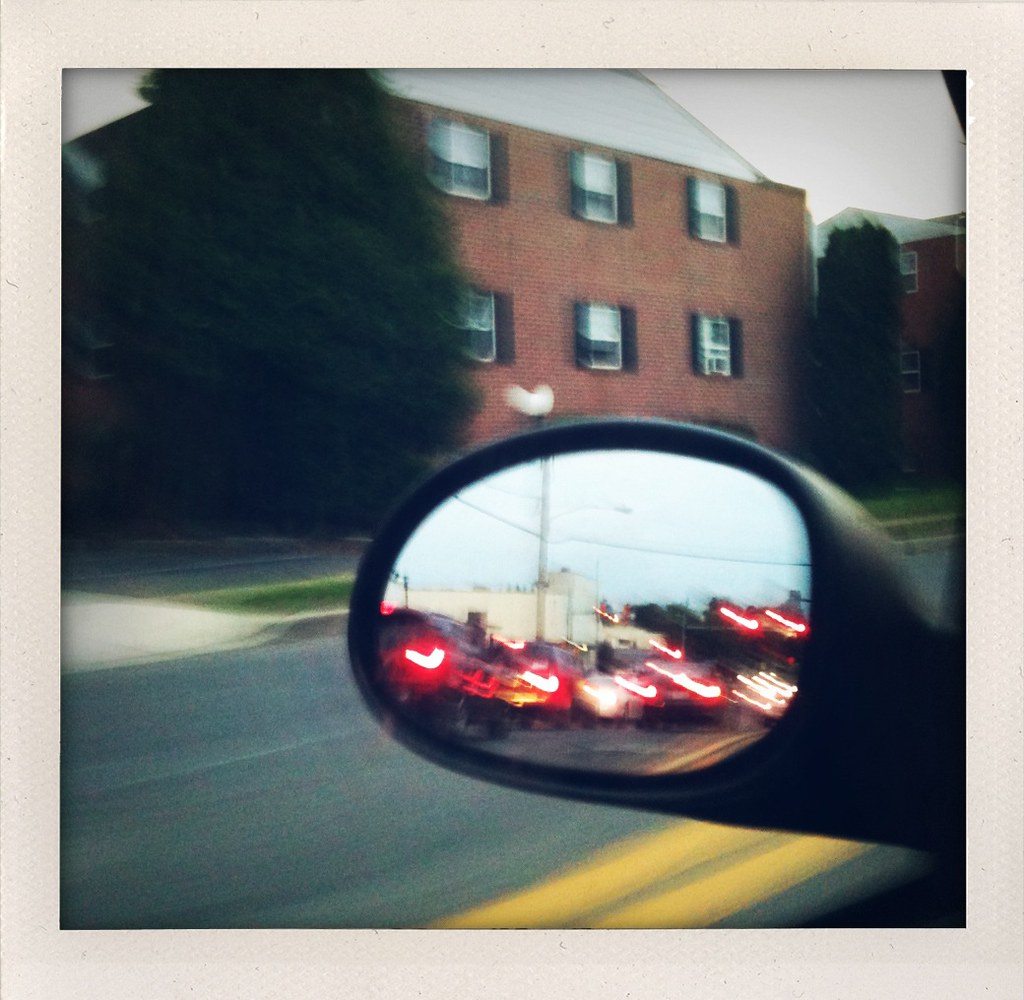The photo is taken from a moving car at dusk, capturing an eclectic mix of urban and vehicular elements. Dominating the left-hand side is the black housing of the car's rear-view mirror, reflecting a montage of blurred vehicles, notably motorcycles with streaking headlights. The mirror also captures a distant white building under a slightly overcast, grayish-blue sky. Below, the rear-view mirror reveals the double yellow lines and the dark gray surface of the road.

Adjacent to the moving vehicle is a sidewalk bordered by patches of green grass and leading to a residential area. Prominently featuring in the scene are two large evergreen trees flanking a red and orange brick building with six windows adorned with black shutters and topped by a white roof. The upper left-hand corner of the photograph is largely occupied by this building and trees, while a similar second brick building appears partially in the upper right-hand corner. The overall scene exudes a residential charm accentuated by the blurred, dynamic atmosphere of the moving vehicles.